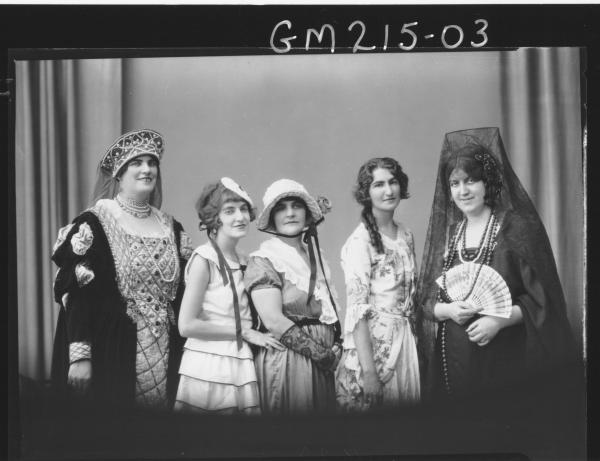The historical black and white photograph labeled "GM 215-03" features five young ladies dressed in various period costumes, standing upright in front of what appears to be theater curtains. The woman on the far left is a heavier set lady adorned in medieval royal regalia, complete with pouf sleeves, a wide hat with a veil, and an abundance of jewels. Next to her is a young lady in a simple sleeveless sundress, accessorized with a flat hat featuring a long ribbon. The third woman, positioned in the center, wears a plain dress with a large bib and a sun hat pulled down on the sides, complemented by lacy black gloves. The fourth lady is dressed in a prairie-style house dress adorned with flowers; she uniquely forgoes headwear, allowing her hair to fall freely in a simple across-the-shoulder ponytail. The woman on the far right, also larger in stature, is draped in a dark gown accented by a Spanish-style veil and elaborate long beaded jewelry, and she holds a hand fan in front of her. Together, their attire suggests they are dressed as historical characters rather than depicting people from the era, adding an air of theatricality to the scene.